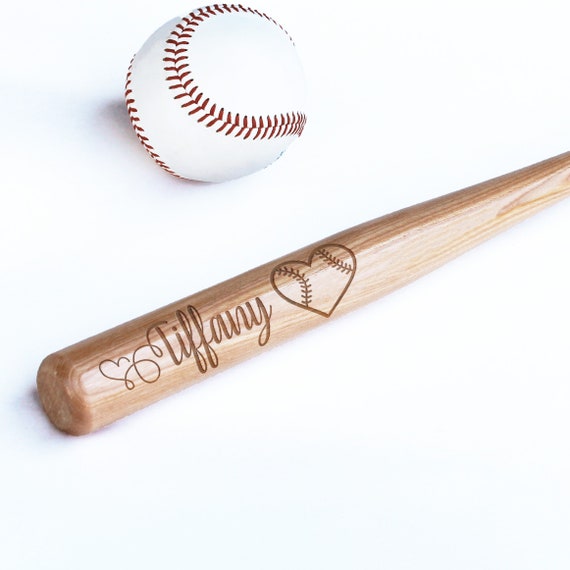The image features a traditional white baseball with red stitching positioned in the top left corner, appearing new and unused. Below the baseball, partially visible, is a pale wooden baseball bat, with about two-thirds of its length extending from the top right to the bottom left of the frame. The bat is intricately engraved with the name "Tiffany" in cursive script. The engraving starts with a heart, followed by decorative curly lines that blend into the "T," and ends with another heart designed with baseball-like stitching. The bottom knob of the bat is cropped out of the image.